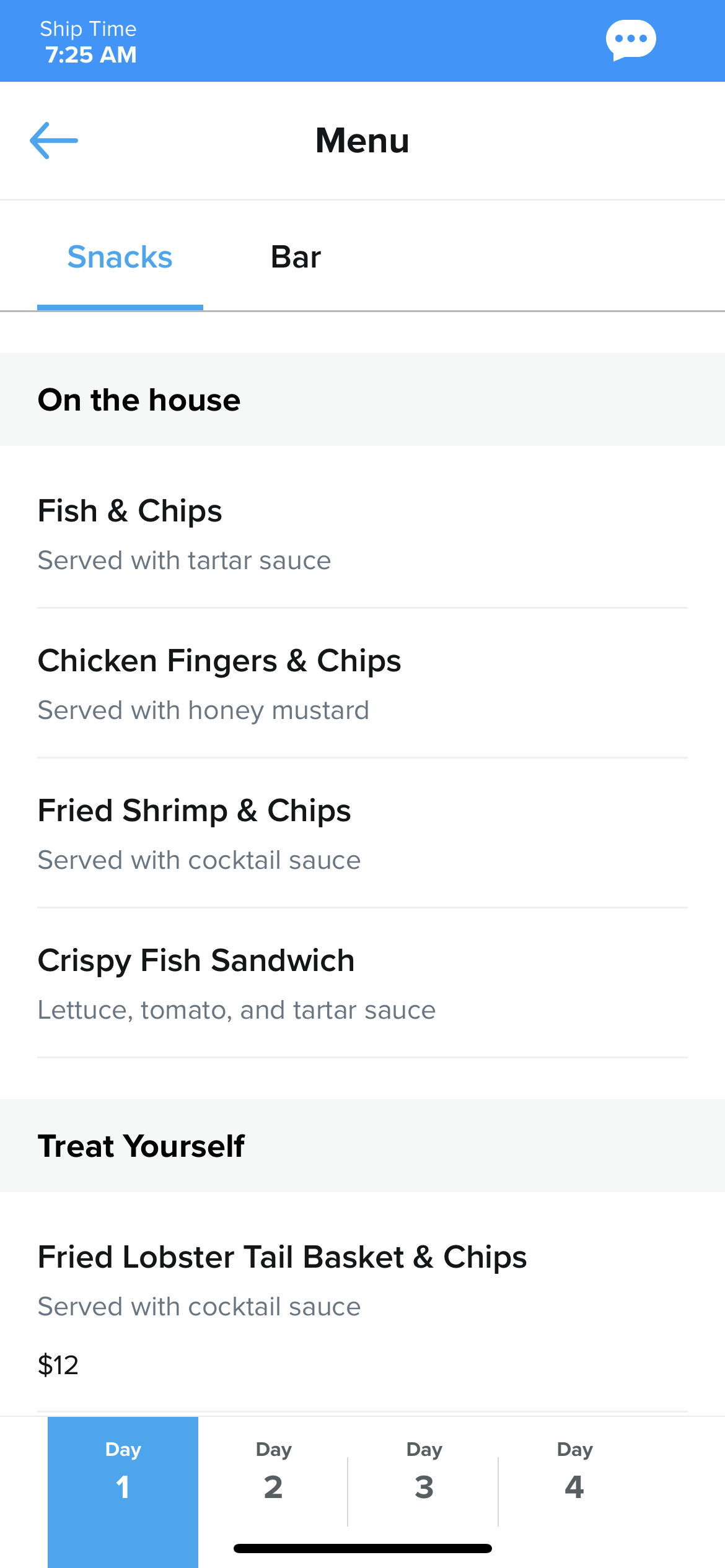Here we have a screenshot of a menu, although the restaurant name is not indicated. At the top of the screen, it shows "ship time, 7:25 AM," along with a message icon. The top part of the menu displays "Menu" prominently and is split into two tabs: "Snacks" and "Bar." The image is focused on the "Snacks" tab.

There are two sections within the "Snacks" tab: "On the House" and "Treat Yourself." Under the "On the House" heading, the following items are listed:

1. **Fish and Chips** - Served with tartar sauce.
2. **Chicken Fingers and Chips** - Served with honey mustard.
3. **Fried Chicken and Chips** - Served with cocktail sauce.
4. **Crispy Fish Sandwich** - Topped with lettuce, tomato, and tartar sauce.

Beneath the "Treat Yourself" heading, the menu features:

1. **Fried Lobster Tail Basket and Chips** - Served with cocktail sauce, priced at $12.

At the bottom of this screenshot, there are four rectangular sections labeled "Day One," "Day Two," "Day Three," and "Day Four." "Day One" is highlighted in blue, while "Day Two" and "Day Three" have bold underlines beneath them.